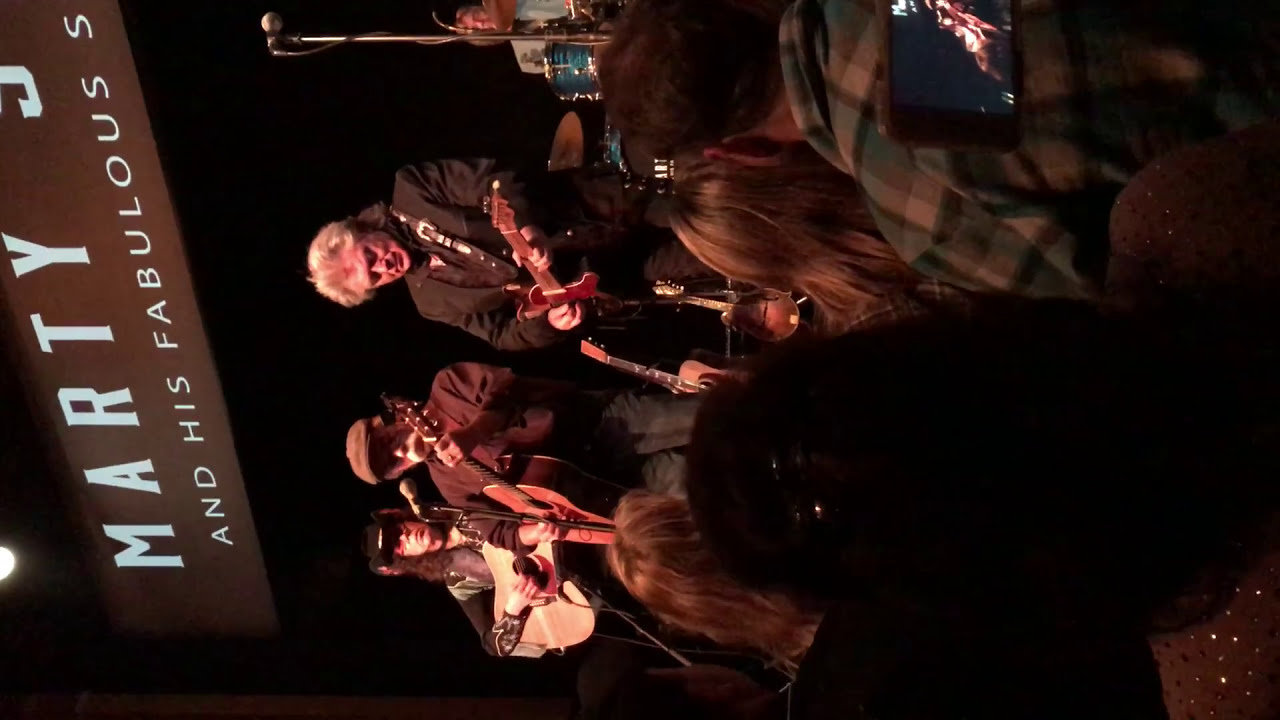In a dimly lit room, the photo shows a slightly rotated scene of a band performing live on stage. The stage is illuminated, emphasizing three musicians playing stringed instruments, including acoustic guitars, with a blue drum set and a glimpse of the drummer's hand in the background. The lead guitarist, distinguishable by his longer gray hair and black suit, appears to be in his 60s and sports a black guitar strap with buckles. Next to him, another guitarist wearing a brown sweater and an English-style cap plays an acoustic guitar. The third guitarist in the back left corner dons a black cowboy hat with a silver strap. Above them, a partially visible brown sign reads "Marty's and his fabulous [unreadable]." In the foreground, several audience members with their backs turned are seated, and a black object, unidentifiable due to its proximity, slightly obstructs the view. A microphone stand is also visible on stage, in front of the drummer.